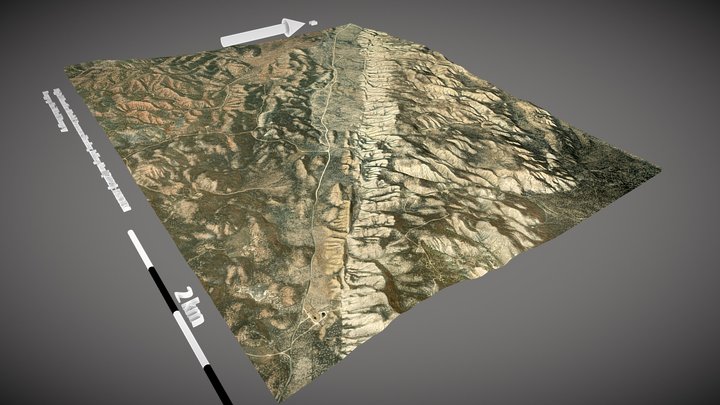This digitally synthesized image depicts a suspended 3D landscape in the shape of a square, floating in space. The landscape predominantly features an arid and mountainous terrain, characterized by extensive reddish and tan-colored regions. Patches of green foliage are evident, especially towards the far left and right edges of the image. 

A notable feature is a linear formation that extends from the bottom middle to the top middle of the landscape, suggesting a geological or topographical division. On the left side of the landscape, there is three-dimensional, white text that is unreadable from the current viewpoint. 

Along the bottom of the suspended land, a white and black striped line is visible, with "two kilometers" inscribed above it in the same three-dimensional white lettering, likely indicating a scale. A white dot, unconnected to the suspended land, appears near the top of the image, highlighted by a 3D arrow pointing towards it from the left side.

The background is a gradient of gray, darker towards the corners, which subtly contrasts with the landscape, providing depth and focus to the central suspended terrain.